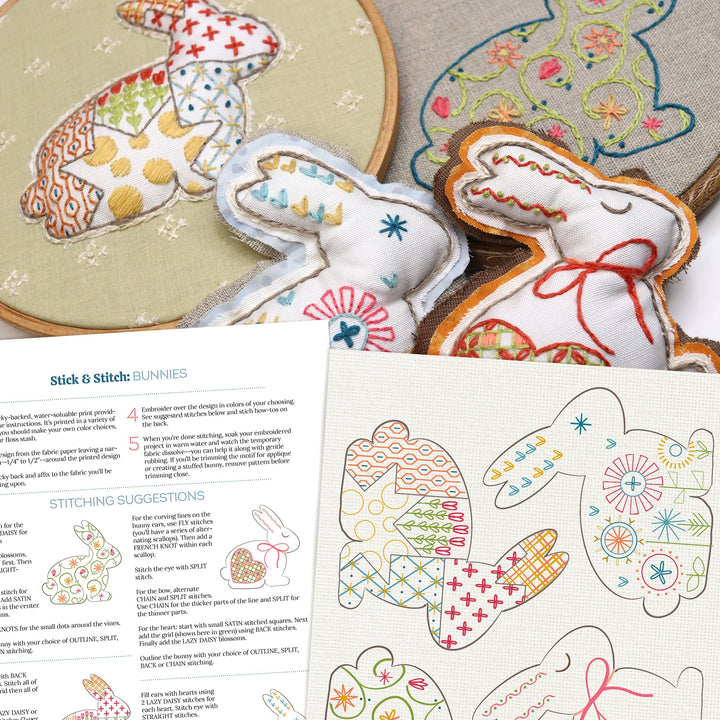The image is a large, detailed promotional banner for an embroidery pattern featuring stuffed rabbit shapes. The top half showcases finished bunnies, intricately embroidered and stuffed, positioned within circular frames with brown wooden borders in the upper left and right corners. The bunny on the left has a gray and white ruffled edge with blue and tan ear decorations and a red, white, and blue circular pattern in the center of its body. The bunny on the right has a brown edge, an orange bow around its neck, and a decorative pattern on its lower half.

In the middle section, partially overlapping the bunnies, is a textured page featuring outlines for four larger rabbit shapes, though only the top two are fully visible. Below this, a white instruction page labeled "Stick and Stitch Bunnies" provides numbered steps and stitching suggestions. The black text offers guidelines for embroidering over the design with colors of one's choosing, along with adjustments and stitch how-tos on the back. The instructions advise soaking the finished project in warm water to dissolve the temporary fabric, with gentle rubbing to aid in trimming the motif. This comprehensive banner elegantly combines visual examples of the finished product with clear, partially visible step-by-step instructions.